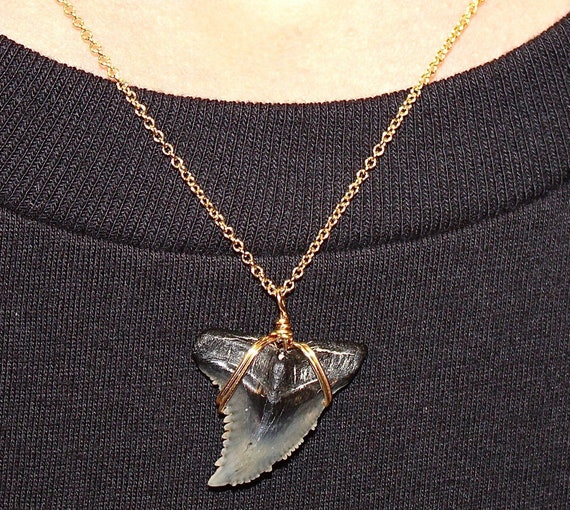The image depicts a close-up shot of a gold chain necklace with a pendant that appears to be a shark tooth. The pendant, which curves to the left and has a jagged, triangular shape, features a combination of black and gray hues—the base is black, and the pointed tip is gray. The tooth is secured to the chain by a tightly wound spiral of gold-colored metal wire that wraps around the upper left and right sides of the tooth. The fine-knit, dark gray sweater of the wearer contrasts with the lighter, peach-colored skin, indicating the wearer has a Caucasian complexion. The sweater has a vertical grain with a distinct lip at the neckline, and the lines of the knit are mostly diagonal near the top. The photograph captures the simple yet elegant design of the necklace and the sharp, intricate details of the pendant, making it a striking focal point against the dark fabric.